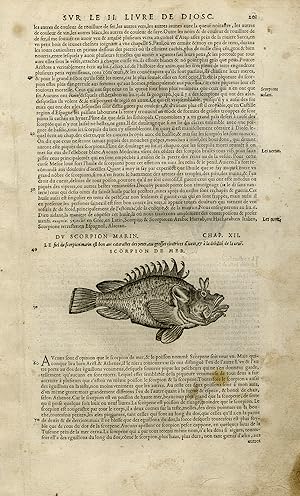This is an illustrated page from an old, slightly dirty book that is not written in English, featuring intricate, hand-drawn artwork and detailed paragraphs. The top of the page prominently displays the text "S-V-R-L-E-L-I-B-R-E-D-E-D-I-O-S-C" repeated twice. This is followed by the number 104, indicating the page number. About two-thirds of the way down, the text "by Scorpion Marin" appears, preceding "CHAP X-I-L," which could potentially denote chapter 49, though the exact meaning is uncertain. Below this chapter heading is another line of text that is unreadable, followed by the words "Scorpion de Mer." The focal point of the page is a meticulously drawn fish with a grotesque appearance. The fish has a jutting bottom lip, an open mouth, and a top jaw diagonally pointing to the right. It features what look like rabbit ears above its eyelids, split fins running down its back forming a C-shape, and dual pairs of dorsal and ventral fins. This monochrome illustration is surrounded by text on both the top and bottom, detailing information about this eerie marine creature referred to as the "Scorpion of the Sea."